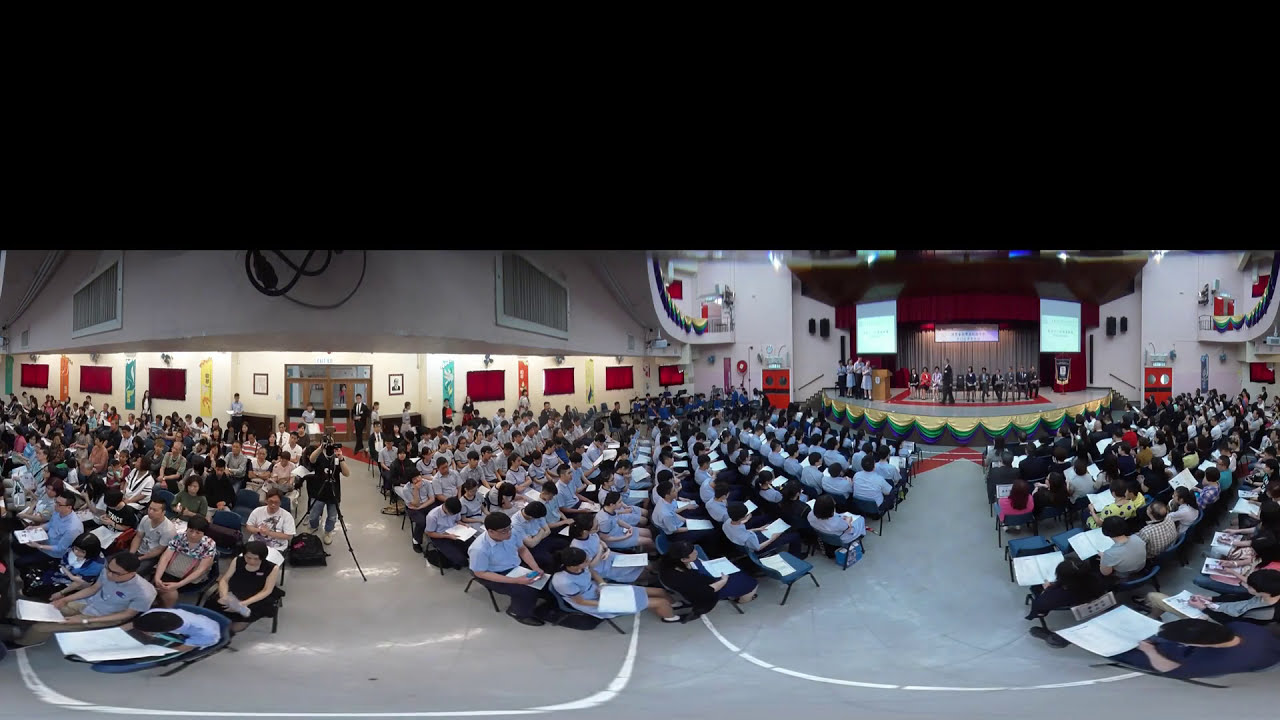The image depicts a large, panoramic view of a bustling auditorium filled with many people, primarily students. The room extends in multiple directions and is arranged in a semi-circular or U-shape formation. The audience members are seated at desks, each with a white piece of paper in front of them, suggesting they might be involved in an activity like taking a test, following a program, or waiting for an event to start. On the stage, located at the far right of the image, people are both sitting and standing, dressed in black, possibly overseeing or presenting something. Several projector screens are also visible near the stage, hinting at an official presentation, conference, or ceremony. The seated audience is mostly wearing matching gray or light blue t-shirts, and many appear to be of Asian or Chinese descent, with dark hair. The auditorium's white walls are adorned with vibrant posters in orange, teal, and yellow, and red decorations that could be windows, flags, or signs. There is a gray curtain behind the stage, enhancing the formal atmosphere of the occasion. Additionally, there are a few individuals, including a cameraman and a person in a suit, suggesting the event's significance might warrant documentation or supervision.